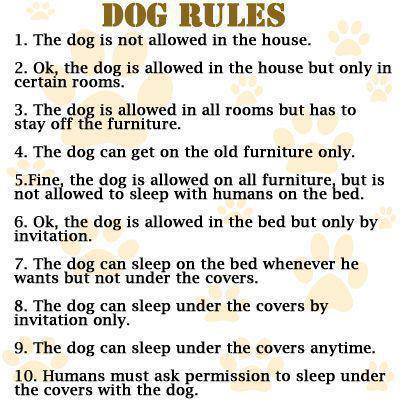This image is a vertical rectangular poster set against a white background. At the top, in bold gold letters, it reads "Dog Rules." Below the title, there are ten humorous rules listed, each progressively loosening restrictions on the dog. The text is written in all capital letters in brown. The rules are as follows: 

1. The dog is not allowed in the house.
2. Okay, the dog is allowed in the house but only in certain rooms.
3. The dog is allowed in all rooms but has to stay off the furniture.
4. The dog can get on old furniture only.
5. Fine, the dog is allowed on all furniture but is not allowed to sleep with humans on the bed.
6. Okay, the dog is allowed in the bed but only by invitation.
7. The dog can sleep on the bed whenever he wants but not under the covers.
8. The dog can sleep under the covers by invitation only.
9. The dog can sleep under the covers anytime.
10. Humans must ask permission to sleep under the covers with the dog.

This poster humorously illustrates the gradual relaxation of rules for the dog, ultimately showing the dog gaining complete control.